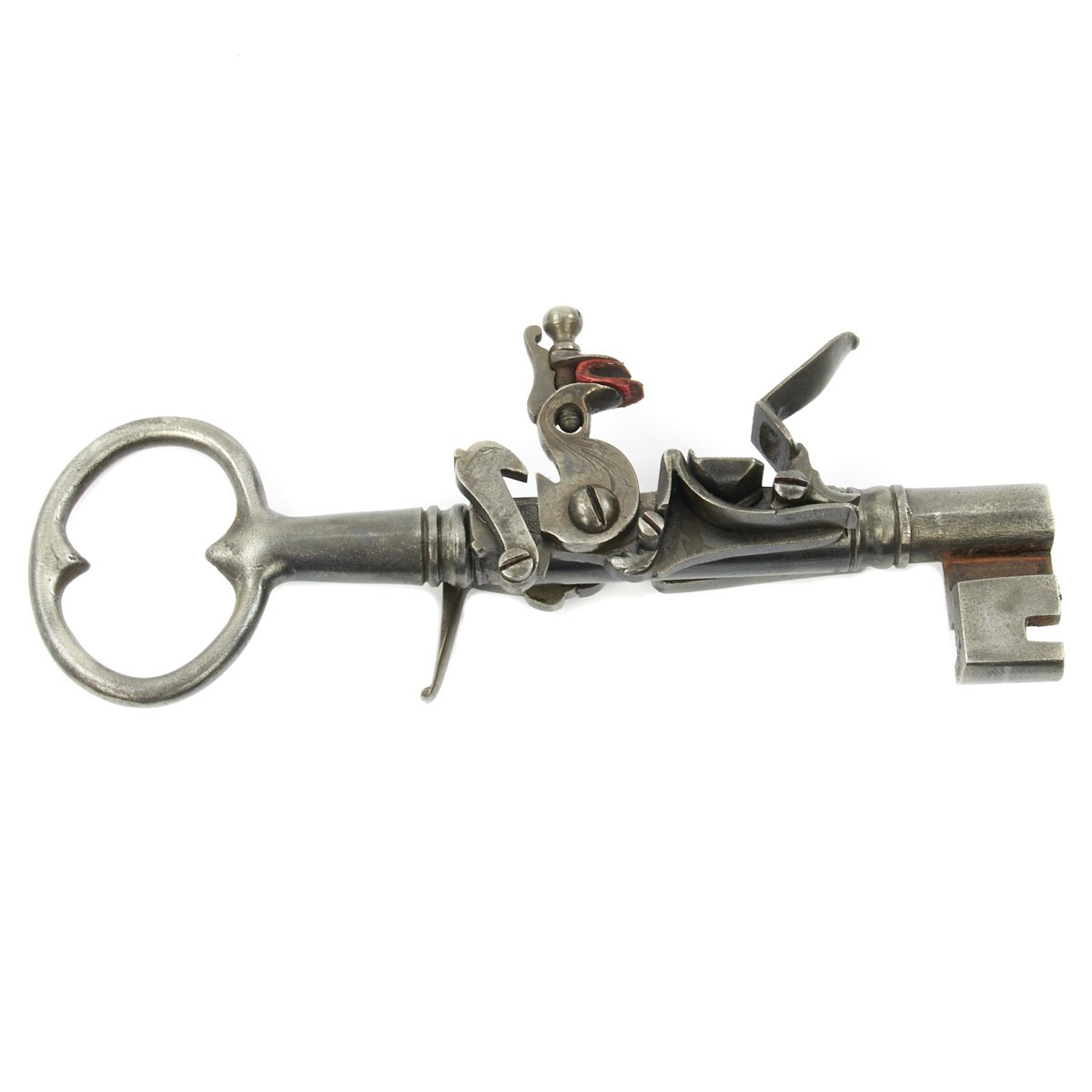This image features a detailed and elaborate mechanical key made of silver metal. The key's head is circular, reminiscent of a bottle opener, allowing it to be threaded through a chain. Extending from the round head, the body of the key is long and slender, adorned with various metal components and screws. Midway down the shaft, several intricate parts and attachments become visible, including a small red section that stands out against the predominantly silver-gray color of the key. One attachment resembles a safety lock, appearing to control the functioning of other components, while another has a bird-like shape. Toward the end, there's a notable rectangular section with a small square cutout, and just above it, a hook-like feature. The very end of the key contains what appears to be a locking mechanism, suggesting it could be used to unlock a door. Overall, this key, approximately five to six inches long, is complex and uniquely designed with multiple moveable parts and connectors.